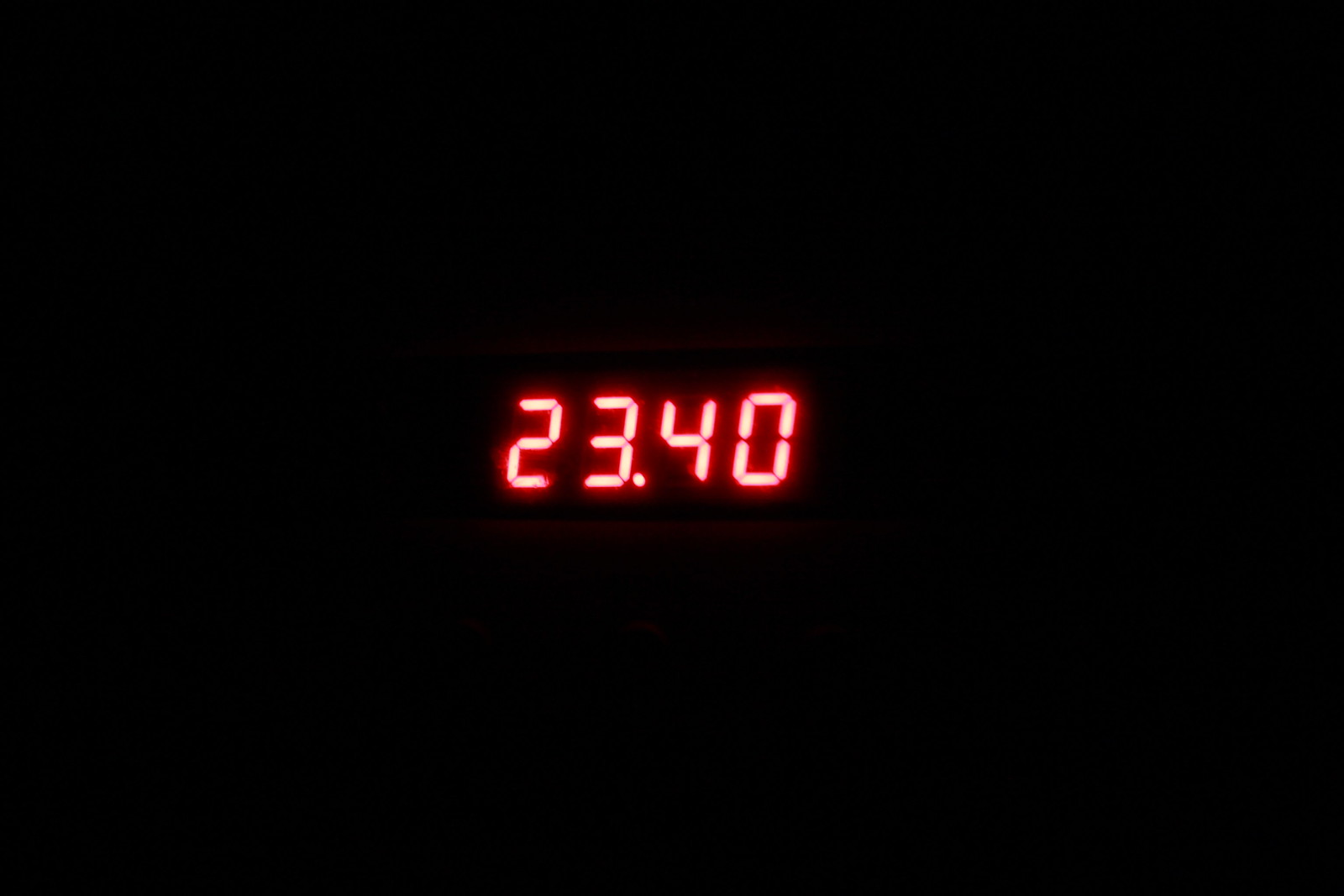In this photograph, set against a simple solid black background, we see an LED display illuminated in a slightly yellow-orange or pinkish red hue. The display reads "23.40" in blocky, segmented digits that are characteristic of LED readouts, with each number formed from a series of straight lines: the 2 and 4 are composed of 4 sections each, the 3 has 5 sections, and the 0 has 6 sections. The digits glow prominently, with their light subtly outlining them in a darker red. This display likely indicates a measurement or numerical value, as it lacks the colon typically seen in clock displays, although its specific purpose remains ambiguous.